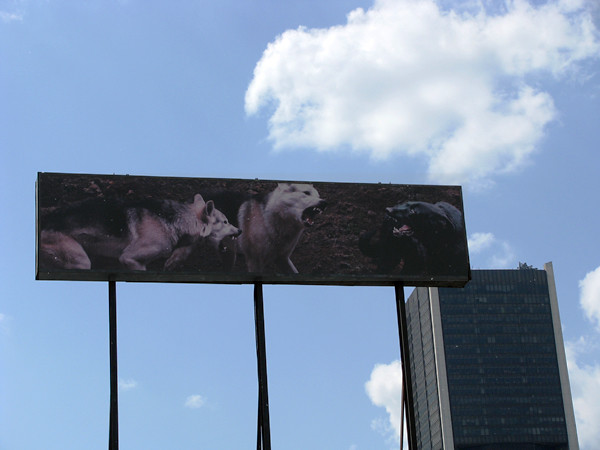The image captures a dynamic urban scene in daylight. Dominating the right side of the photo is a tall skyscraper-style building with a predominantly dark gray facade and white trim. On the left side, a large billboard is elevated by three tall, black poles. The billboard prominently features an image of three wolves, with the leftmost wolf displaying a gray and white coat, the center wolf also gray and white, and the rightmost wolf appearing black. All three wolves have their mouths wide open, revealing their canines, suggesting a scene of aggression or fighting. The background shows a light blue sky with puffy white clouds scattered throughout, adding contrast to the otherwise detailed and intense foreground elements.